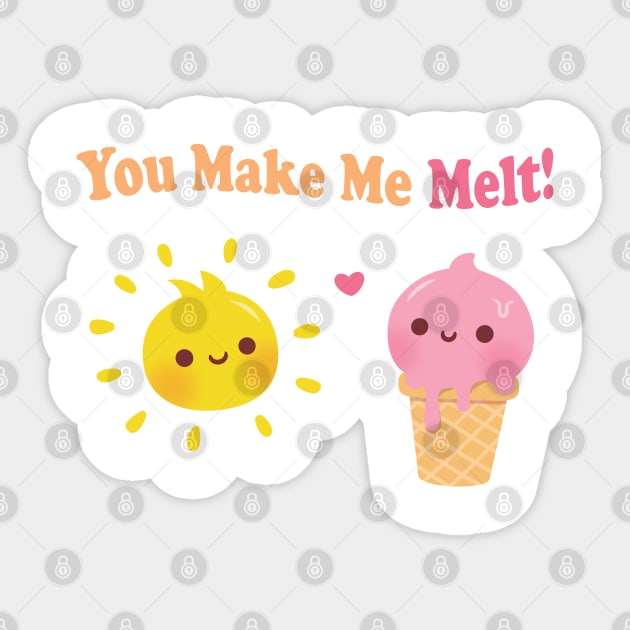This image is an illustrated drawing featuring a cartoon-style sun and an ice cream cone, both with expressive eyes and mouths depicted in black. The sun, located on the left side of the drawing, is yellow, while the ice cream cone on the right is brown with purple ice cream. Above these characters, a playful message reads "You make me melt" with "you make me" written in brown and "melt" in purple.

The illustration is enclosed within a white, cloud-like shape, with the rest of the background being light gray and adorned with a pattern of small diamonds. Each diamond has a circular watermark of a lock at its center.

A small heart in pink is situated between the sun and the ice cream cone, adding to the cute, romantic nature of the illustration. The overall aesthetic suggests it could be a design for a sticker or similar decorative item.